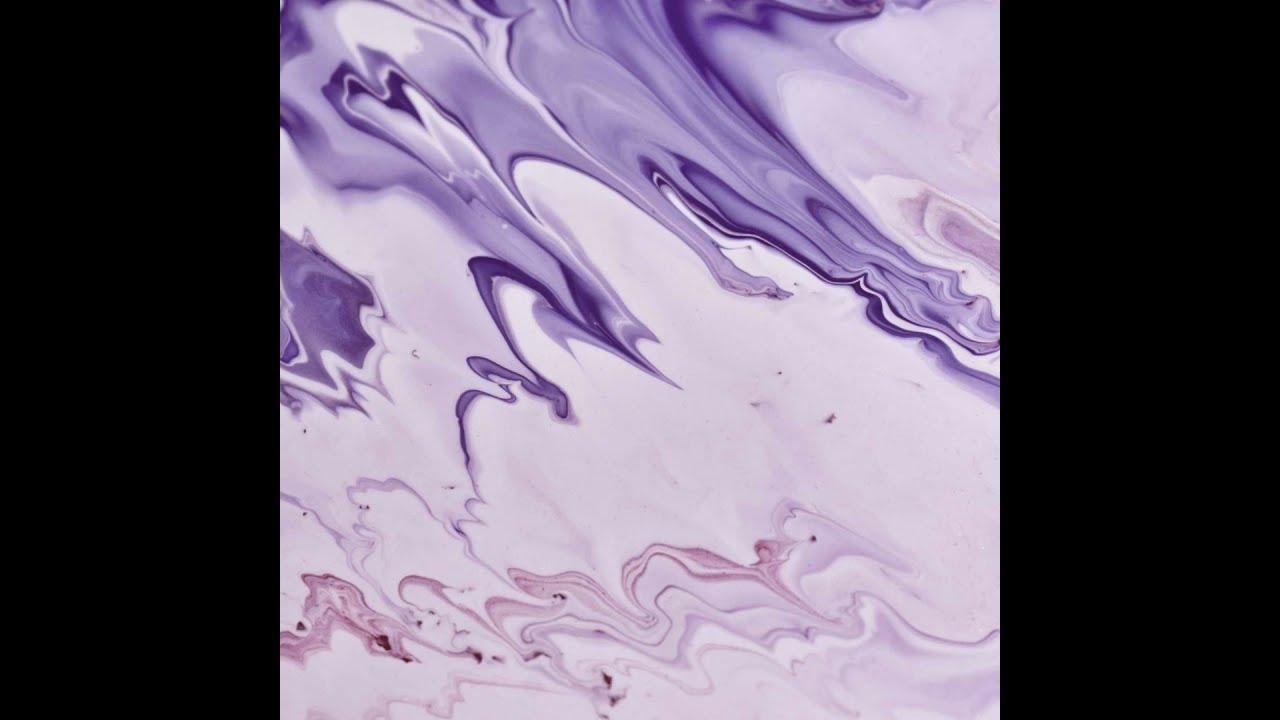The image features an abstract marbled pattern centered within black rectangular borders on the left and right sides. The marbled artwork itself is square-shaped, dominated by swirling hues of purple, pink, and white, creating an effect reminiscent of an oil painting. The background of the marbled area is a very pale pink. Toward the top left corner of the piece, the purple is more concentrated, forming deep, mini peaks that stretch diagonally upwards to the top right corner, where the shade transitions into pink. The pink hue then takes over the bottom half of the image, appearing more subtle and fluid, mixed with white and occasionally highlighted by dark markings. The entire composition creates a jagged, yet fluid appearance, like a geode or mineral rock formation, with some areas displaying pronounced swirls and others almost flat and devoid of texture.